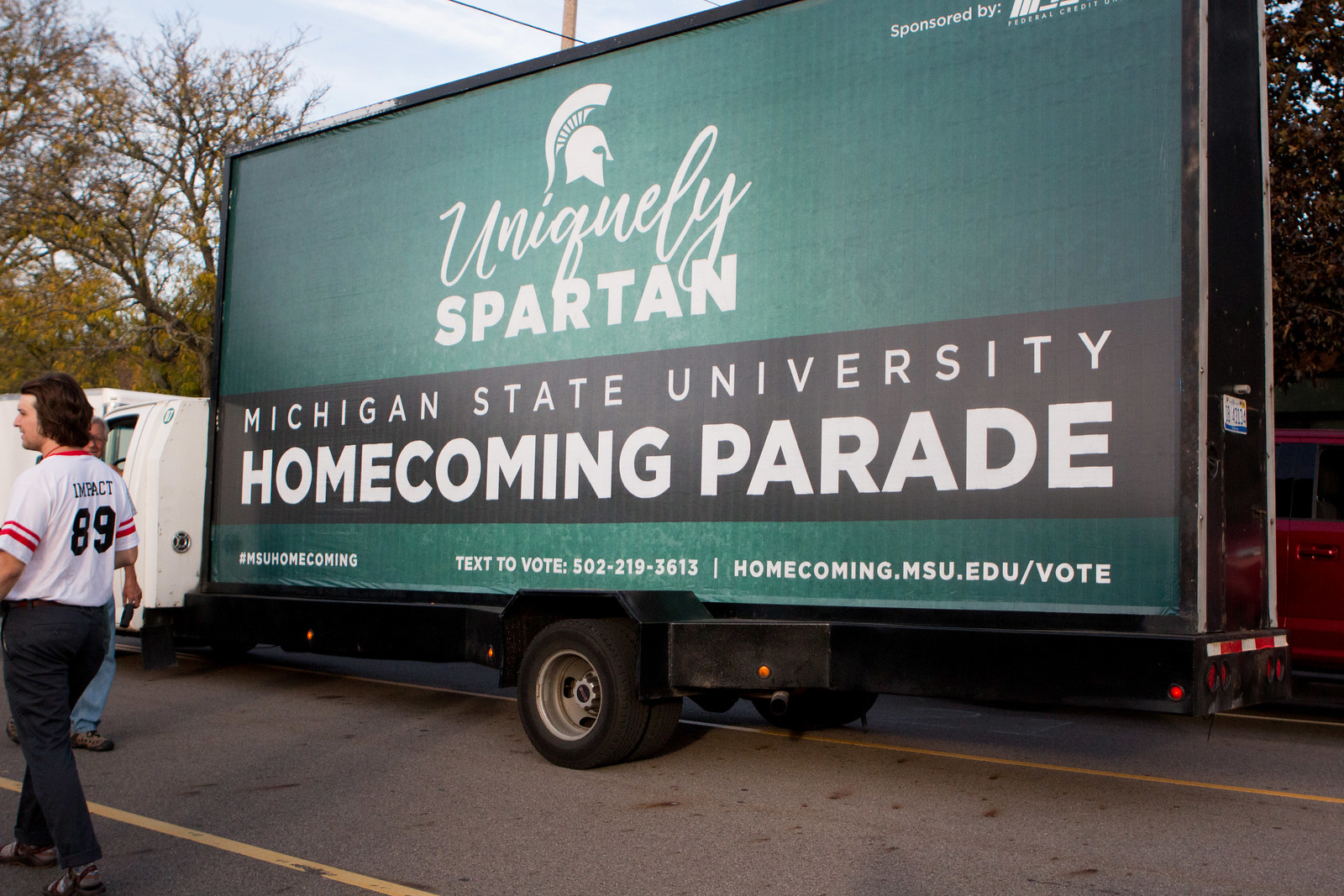The image showcases a thin, white advertisement truck prominently featuring a large, billboard-sized sign with a vibrant dark green background. This sign promotes Michigan State University's Homecoming Parade, with the slogan "Uniquely Spartan" and a Spartan helmet logo. Below this, text in white reads "Michigan State University Homecoming Parade," followed by "Hashtag MSU Homecoming," "Text to vote: 502-219-3613," and "homecoming.msu.edu/vote." The advertisement occupies the entirety of the truck bed, which is black. The scene is set in what appears to be a parking lot, with autumnal trees visible in the background, indicated by the absence of leaves. To the far left of the photo, a person with brown hair, dressed in black pants and a white jersey-style shirt with red trim, labeled "Impact 89" on the back, can be seen.